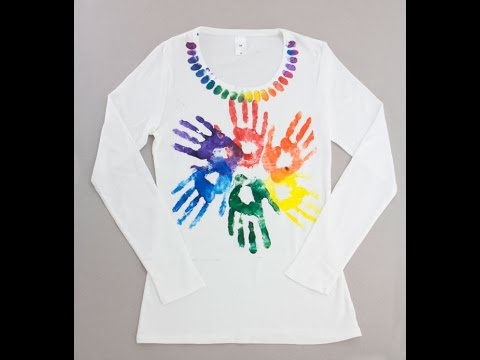This is an image of a handmade, white, long-sleeved t-shirt lying on a grayish-beige background, bordered by vertical black bars on the left and right sides. The shirt is arranged with its sleeves folded inward, resting on the torso. The neckline is adorned with thumbprints in a rainbow of colors: starting from purple on the left, transitioning through blue, green, yellow, orange, and red, and returning to purple on the right. The main artwork on the shirt features six handprints, each representing different colors of the spectrum—red, orange, yellow, green, blue, and violet—radiating outward from the center of the chest in a radial pattern, akin to a rainbow. The handprints are detailed, showing all five fingers, creating a vibrant, artistic display.